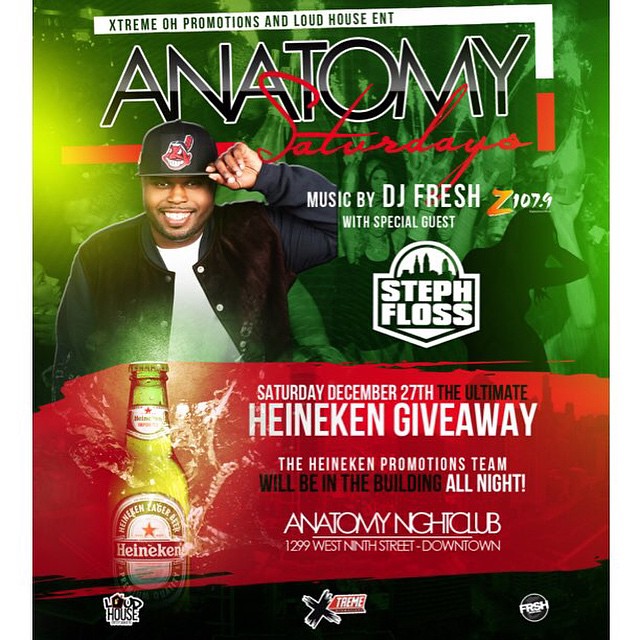This vibrant and colorful poster promotes an event at Anatomy Nightclub. The design features a background that transitions from green to red to black, with images of people dancing and partying. At the top, in a small white strip, the text reads "Extreme OH Promotions and Loud House ENT." Below this is the headline, "Anatomy Saturdays," where "Anatomy" is written in bold black and white, and "Saturdays" is in red cursive. Featured prominently is a black man wearing a Chiefs baseball cap, a black jacket with blue sleeves, and a white t-shirt. He is smiling at the camera and holding the cap with his left hand. The advertisement informs that the music will be provided by DJ Fresh from Z107.9, with special guest Steph Floss. This information is presented inside a logo featuring a city skyline in green. Further down, there is an image of a Heineken bottle with the text, "Saturday, December 27th, the ultimate Heineken giveaway," indicating that the Heineken Promotions team will be in attendance all night at Anatomy Nightclub, located at 1299 West 9th Street, Downtown. Along the bottom, the logos for Loud House, Extreme, and FRSH are displayed.